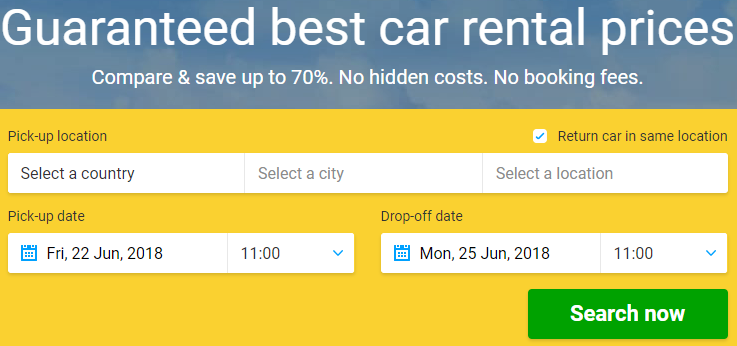This horizontally rectangular image is a screenshot from an unidentified car rental company's website. A light blue horizontal banner spans the top section, prominently displaying "Guaranteed Best Car Rental Prices" in a large, light font. Just below this text, in smaller font, is the phrase "Compare and save up to 70%. No hidden costs, no booking fees."

The main portion of the image has a yellow background with various white boxes overlaid, organizing the rental information. On the left side, the section labeled "Pickup Location" features drop-down menu options for "Select a country," "Select a city," and "Select a location." To the right, there is a checkbox labeled "Return car in same location," which is currently checked.

Beneath the pickup location options, there are fields for the "Pickup Date," set to Friday, 22nd June 2018, at 11:00 AM. Similarly, the "Drop-off Date" is specified as Monday, 25th June 2018, also at 11:00 AM.

At the bottom right corner of the image is a large green "Search Now" button, inviting users to proceed with their car rental search.